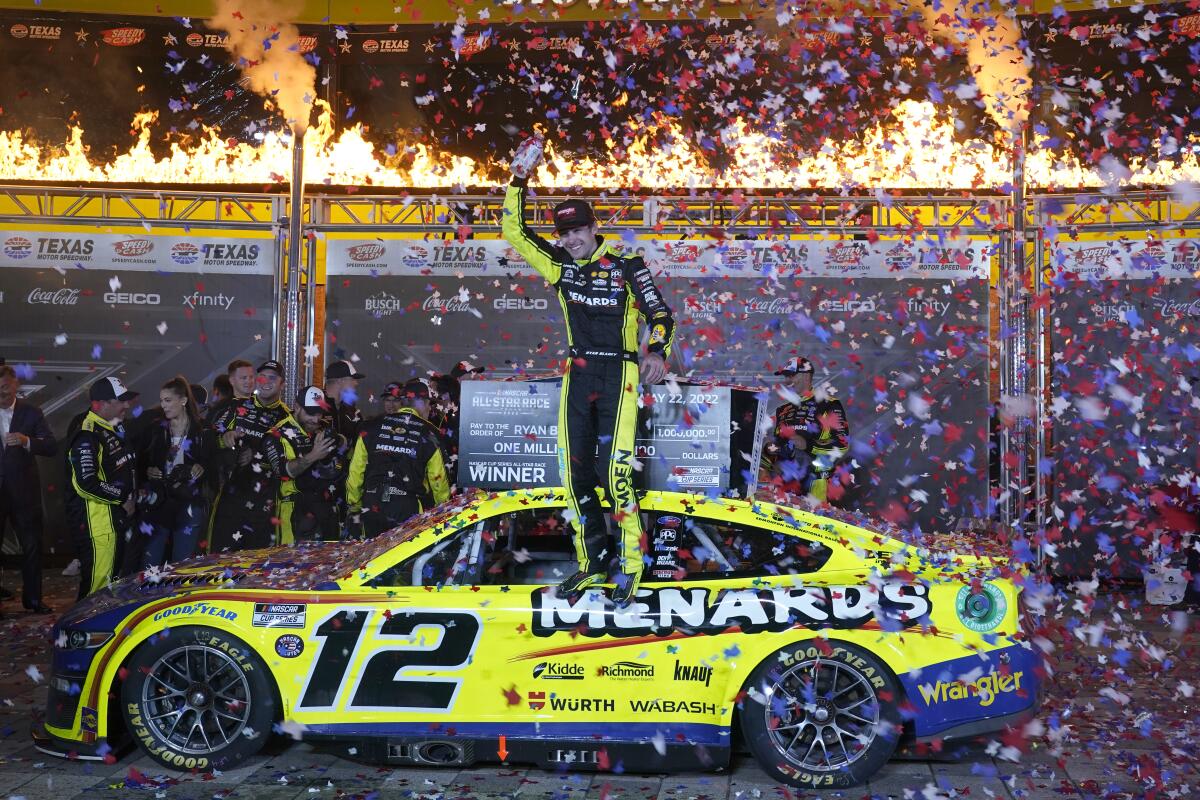In a vibrant and exuberant scene of triumph, a young race car driver named Ryan, likely in his thirties, stands victoriously on the ledge of his driver’s side window. Dressed in a black and yellow jumpsuit adorned with numerous logos, including prominent sponsors like Menards, Goodyear, Wrangler, Wabash, Richmond, and Kidd, he radiates joy, his black hat perched proudly on his head. Ryan holds a beer can in one hand and raises his other in celebration. His predominantly yellow race car, marked with the number 12 and intricate navy blue trimming, sits below him, its surface covered in a mosaic of sponsorship logos. Around Ryan, colorful confetti fills the air as fireworks ignite at the top of the promotional boards behind him, enhancing the celebratory atmosphere. The backdrop showcases a partially obscured check bearing his first name, awarded for an all-star race on May 22, 2022, with a prize of $1,000,000. Flanking the scene, crew members in matching black and yellow jumpsuits share in the jubilation, completing this electrifying snapshot of a NASCAR victory.